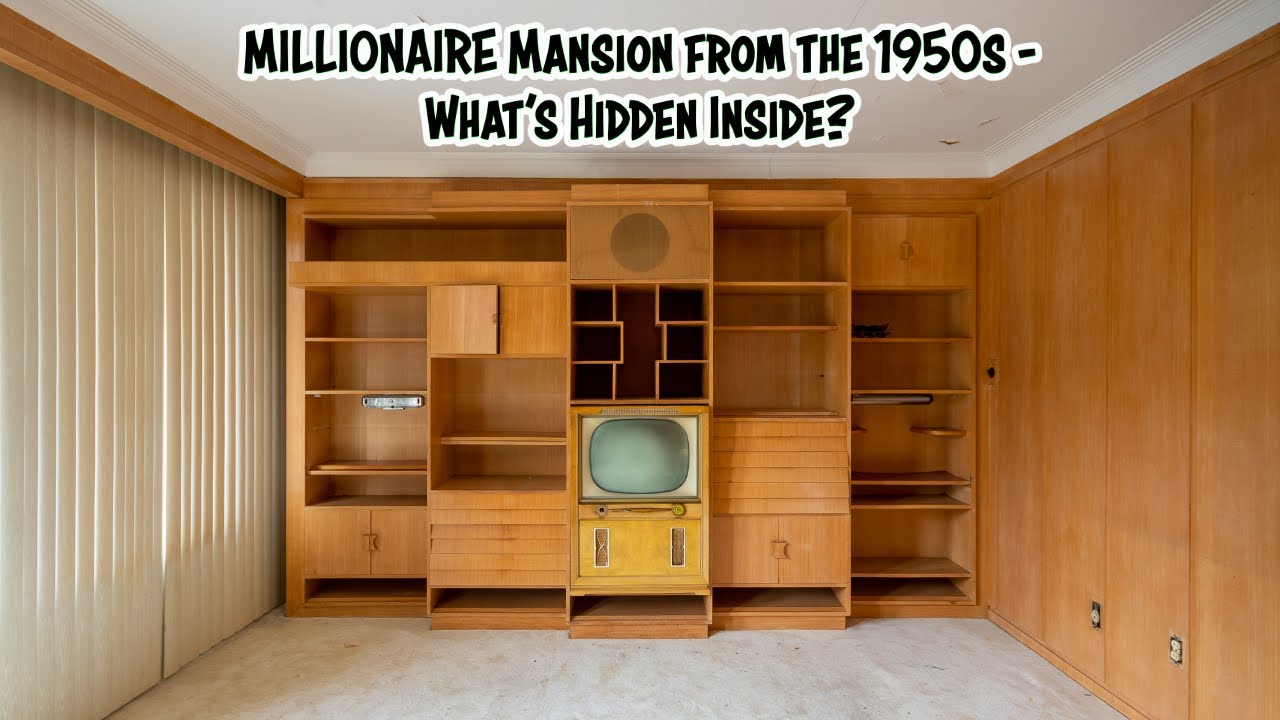The image depicts a cozy living room area in a home, centered around an extensive light brown wooden entertainment center that spans the entire back wall. This entertainment center features numerous empty shelves, offering ample space for storage or display. To the left, off-white mini blinds are fully closed, providing a sense of privacy. The lush, off-white carpet adds a plush, comfortable feel to the room. On the right side of the image, the wall further emphasizes the wooden theme of the entertainment center, blending seamlessly with its design. The overall ambiance suggests a warm and inviting space, perfect for relaxation and entertainment.